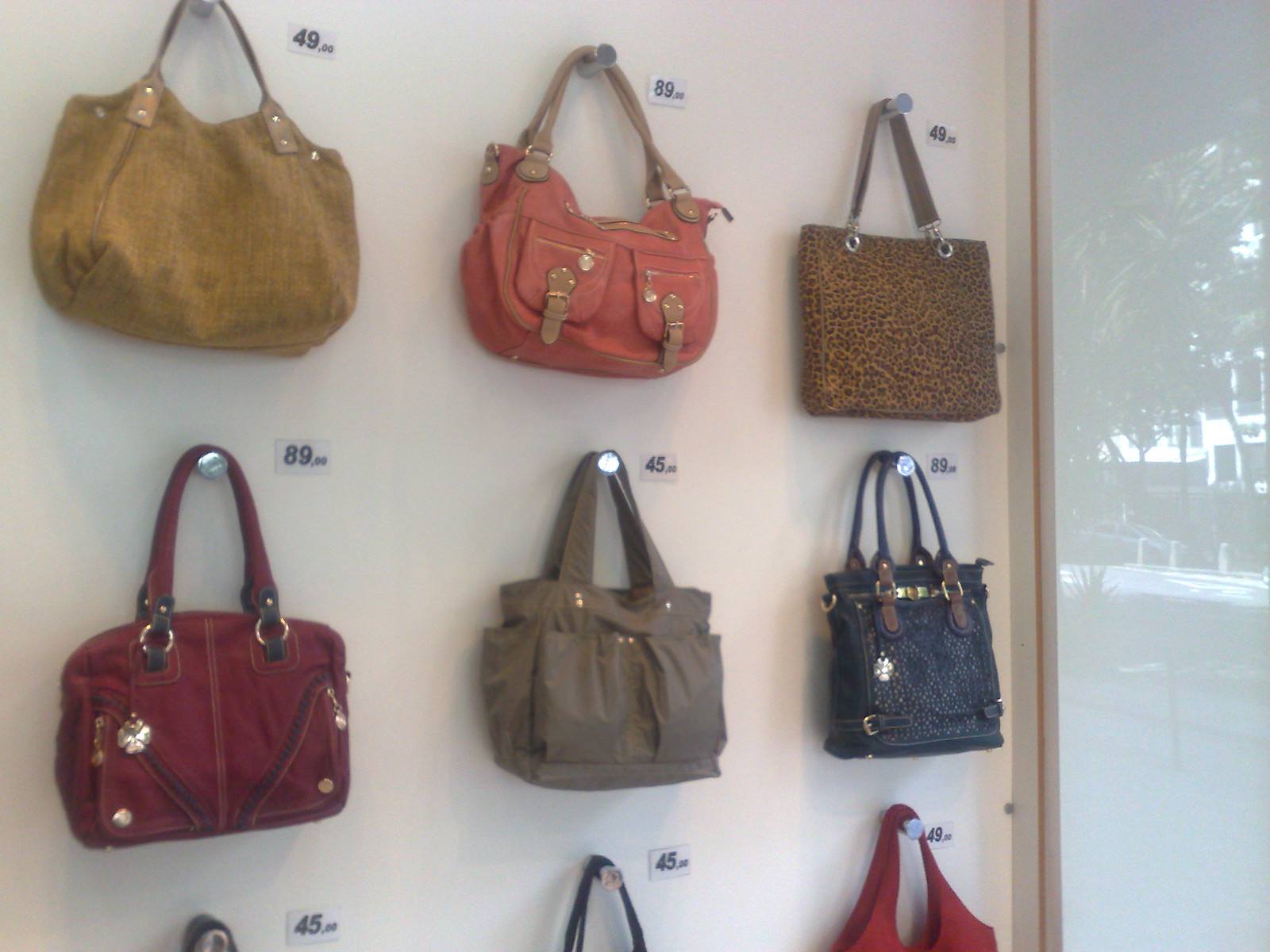This photograph depicts a collection of designer handbags hanging on silver pegs against a white wall. Adjacent to the right of the white wall is a window through which trees and buildings can be seen, adding a touch of greenery and an urban backdrop to the scene. The shot prominently features six full purses and just the straps of three additional purses at the bottom, partially cut off by the edge of the image.

From left to right:

1. The top left bag is tan (described by some as brown or a yellow-greenish shade) and is priced at $49.
2. To its right is a pink purse with two pockets and a brown strap, marked at $89.
3. Next is a square, leopard-print purse, also priced at $49.
4. Below these, the first purse is a dark red handbag with several zipper pockets, priced at $89.
5. Adjacent to it is a dark grey purse featuring loose open pockets, priced at $45.
6. The last fully visible purse is dark blue, embellished with silver and gold straps, and fairly square in shape, though its price appears faded but was noted to be $89 previously.

Each purse has a numbered price tag in the upper corner, and the three handbags at the bottom show only portions of their handles, indicating they are partly out of the frame. The overall setting suggests an organized retail display or an exhibit showcasing these fashionable items.